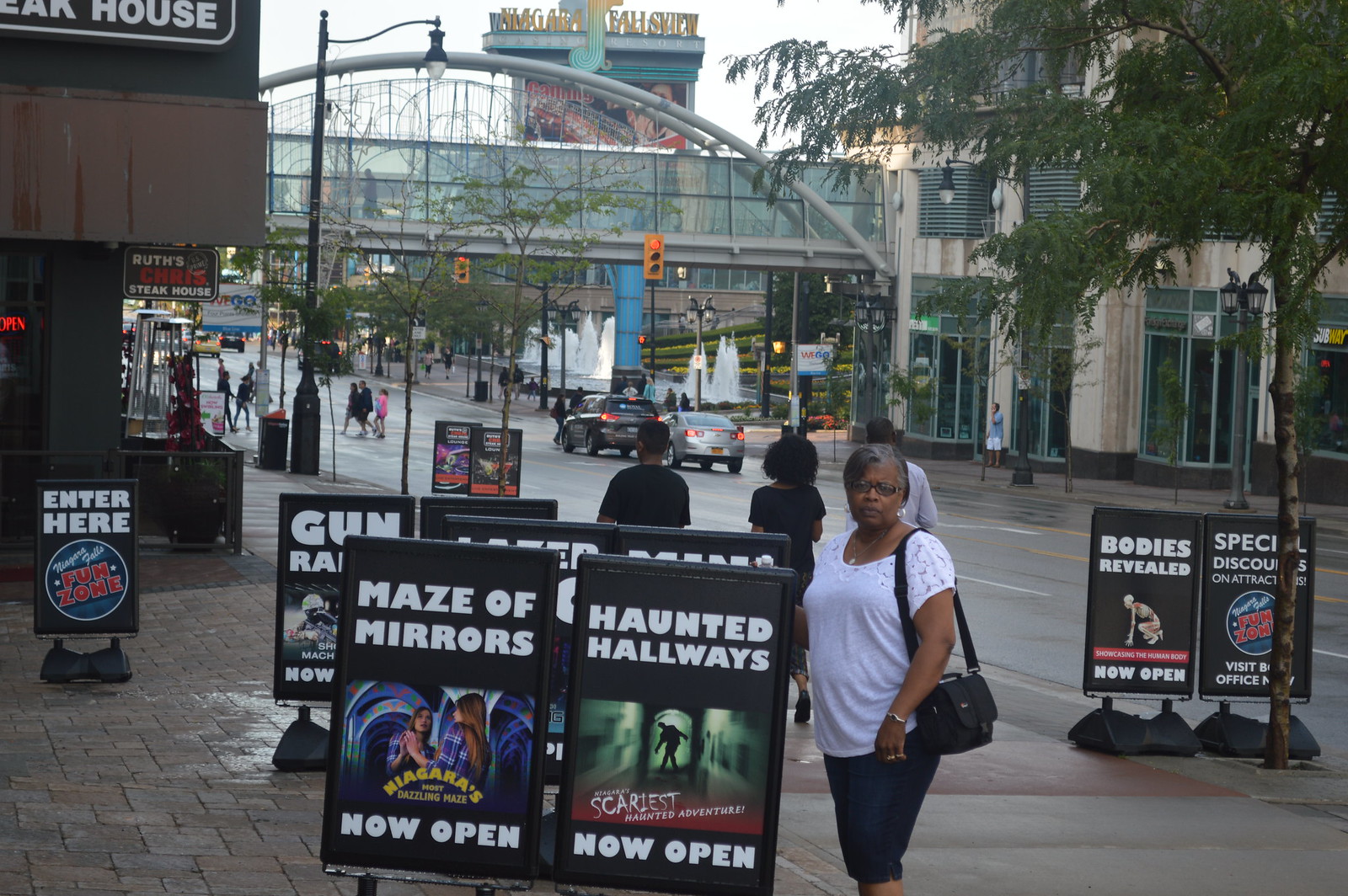In this bright, color photograph set against an urban backdrop, an African-American woman wearing a white short-sleeved shirt, crop pants, and a black shoulder bag poses on a bustling city sidewalk. She stands prominently beside several black signboards with white and red text. The sign to her left reads "Maze of Mirrors - Now Open" while the sign to her right announces "Haunted Hallways - Now Open." Additional signs around her include "Bodies Revealed - Now Open," "Special Discounts - Visit the Office," and "Enter Here - Fun Zone," the latter of which features "Fun Zone" in striking red letters. Behind her, you can spot the sign for "Ruth's Chris Steakhouse," where "Chris" is highlighted in red and the remaining text is in white on a black background. The image captures a busy street scene with pedestrians, cars, palm trees, traffic lights, and a high-rise building in the distant background, giving a lively atmosphere to this Niagara Falls location. The photograph is an example of representational realism, vividly showcasing both the woman and the surrounding commercial environment.